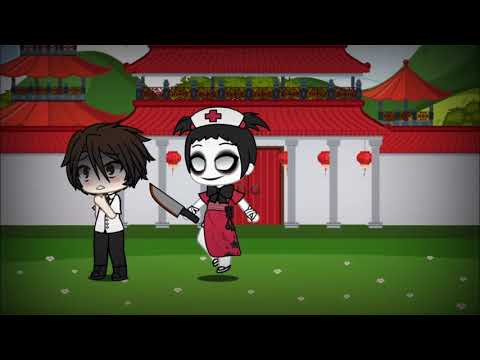This cartoon image depicts an eerie scene featuring oversized, Japanese-style dolls. The focal point is a girl in a nurse outfit, characterized by her ominous, pupil-less grey eyes and black pigtails. She wears a red dress marked with splotches and a white nurse hat bearing a red cross. Floating slightly above the ground, she menacingly points a sharp knife towards a distressed boy with dark, spiky hair. The boy, dressed in a white shirt and black pants, has his hand up to his throat and is facing away from the nurse. They stand in front of a temple-like structure with white walls, red accents, and a red roof, decorated with Japanese lanterns hanging from the columns. The background includes glimpses of green trees, adding to the scene's eerie atmosphere.